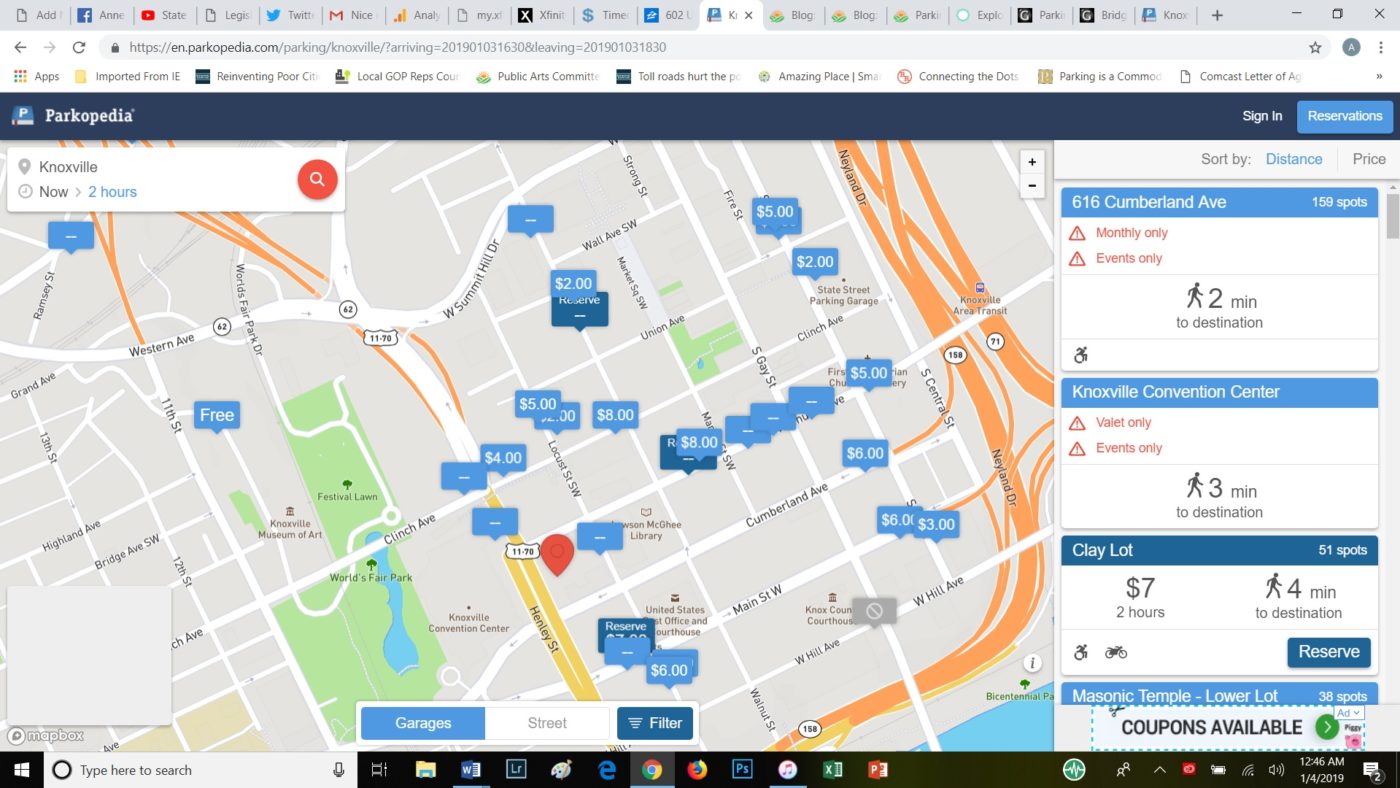A screenshot of a web page depicting someone using Parkopedia to search for parking options in Knoxville. The browser displays numerous tabs open at the top, suggesting a busy multitasking session. The main section of the webpage features an interactive map of Knoxville, highlighted with various parking locations indicated by rectangles containing prices such as $2, $5, and $8. These prices seem to denote the cost of parking in respective areas. 

The user interface includes options for filtering by garages and street parking and a sign-in section for users, possibly for account management or reservations. The page specifically details a location at 616 Cumberland Avenue, noting it is a two-minute walk to the Knoxville Convention Center. For another location named "Clay Lott," it informs users that there are 51 available spots priced at $7 for two hours, with a walking distance of four minutes to the destination. Additionally, there is a clickable link indicating the availability of coupons, potentially offering discounts or special parking rates.